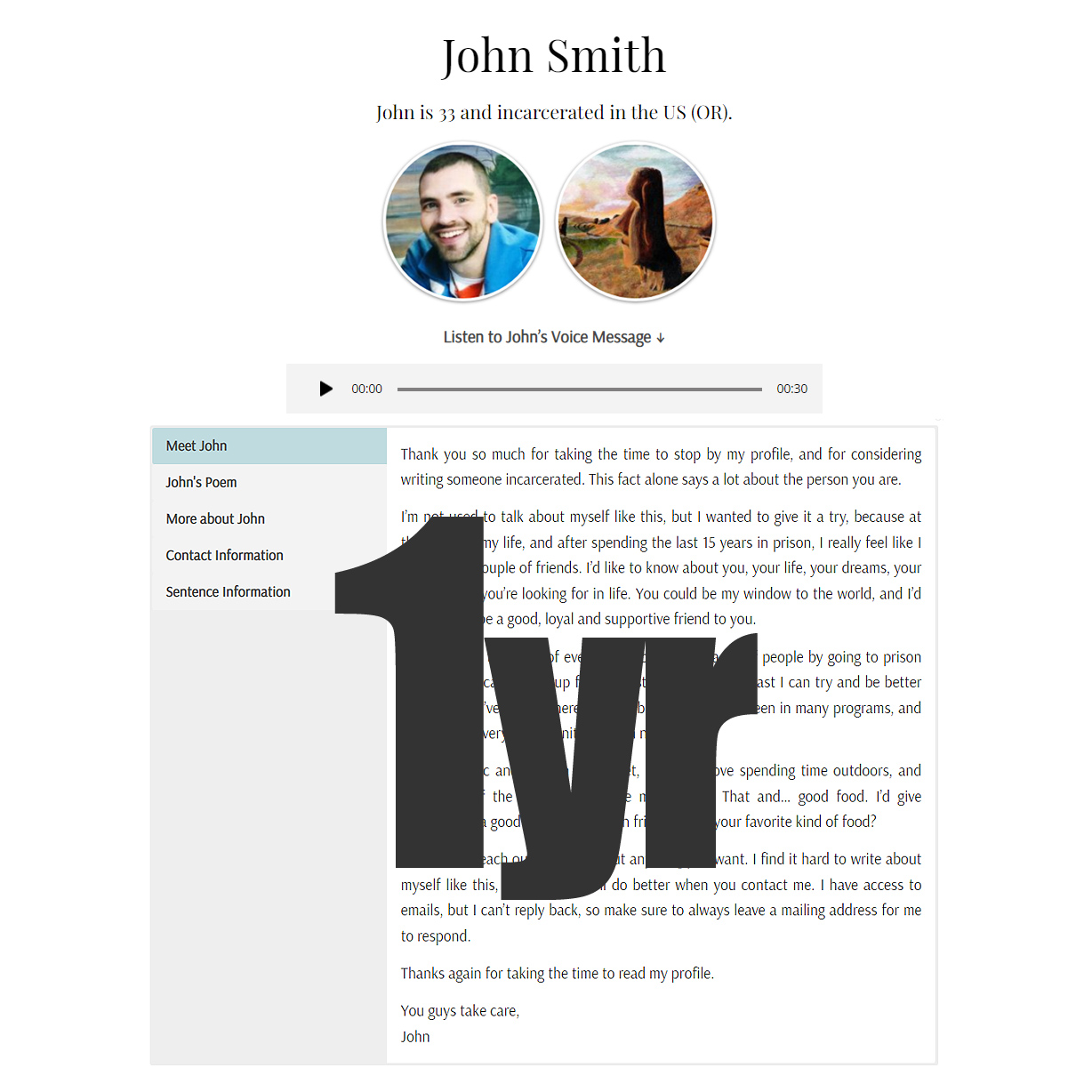This image appears to be a screenshot from a prison pen pal website. At the top, the name "John Smith" is prominently displayed. Below that, it states, "John is 33 and incarcerated in the U.S. (OR)," indicating he is in Oregon. Two circular images are positioned beneath this text; the left one likely shows a picture of John Smith, while the right one features an image reminiscent of the large stone figures found in the Galapagos Islands.

Following these images, there is a prompt inviting users to "Listen to John's voice message," accompanied by a play button to hear the recorded message. On the lower left side, there are links labeled "Meet John," "John's Poem," "More About John," "Contact Information," and "Sentence Information." Next to these links, on the right side, there is a detailed section where John shares information about himself, labeled "Meet John." However, this text is partially obscured by an overlaid large number "1" and the letters "YR," making much of the content illegible.

Overall, the image seems to depict an individual's profile on a platform designed to connect incarcerated individuals with pen pals, providing various ways to learn about and potentially communicate with them.